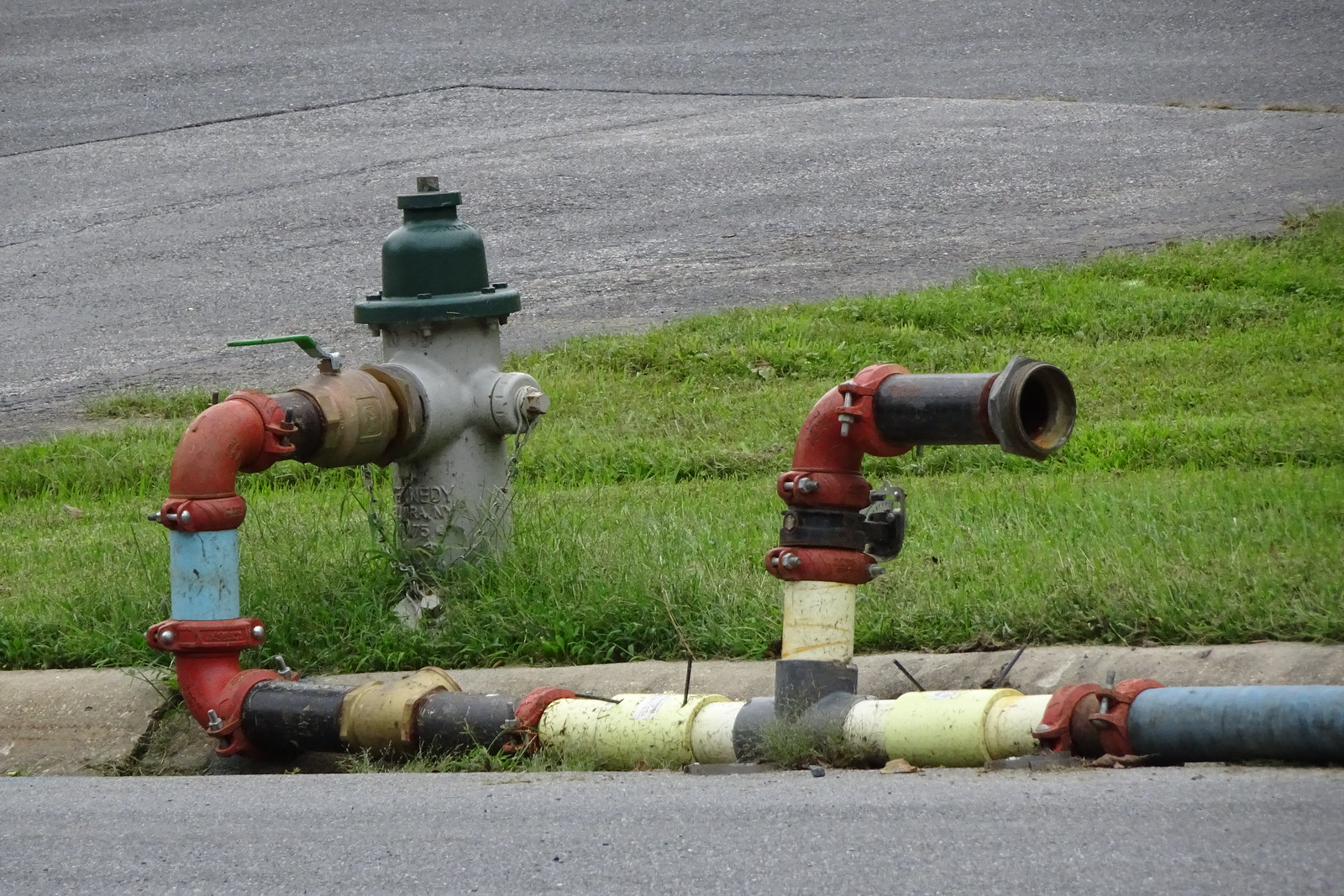The image is a color photograph in landscape orientation, featuring a peculiar fire hydrant setup. At the top of the image, asphalt pavement is visible, with a stretch of green grass occupying the middle section. Toward the bottom, the scene transitions to a curb, concrete curbing, and more asphalt pavement in the foreground. 

The centerpiece is a gray fire hydrant with a green top, which includes rivets on the green knob and cover. Extending from the hydrant is an unusual and motley assortment of pipe segments and couplings. The pipes connecting to the hydrant are of various short lengths and colors, including red, blue, black, gold, brown, and a very light orange. This haphazard assembly includes multiple elbows, sections of pipe, and couplings, suggesting a makeshift construction due to the absence of a long, continuous pipe.

The pipe segments form a somewhat zigzag pattern reminiscent of a caterpillar, leading to a T-shaped section several feet down. This T-section features additional pipes protruding and more elbows, indicative of a complex, improvised setup possibly intended to channel water, though its exact purpose is unclear. The fire hydrant and its extension rest on the green grass, adding to the quirky and ad hoc nature of the scene.